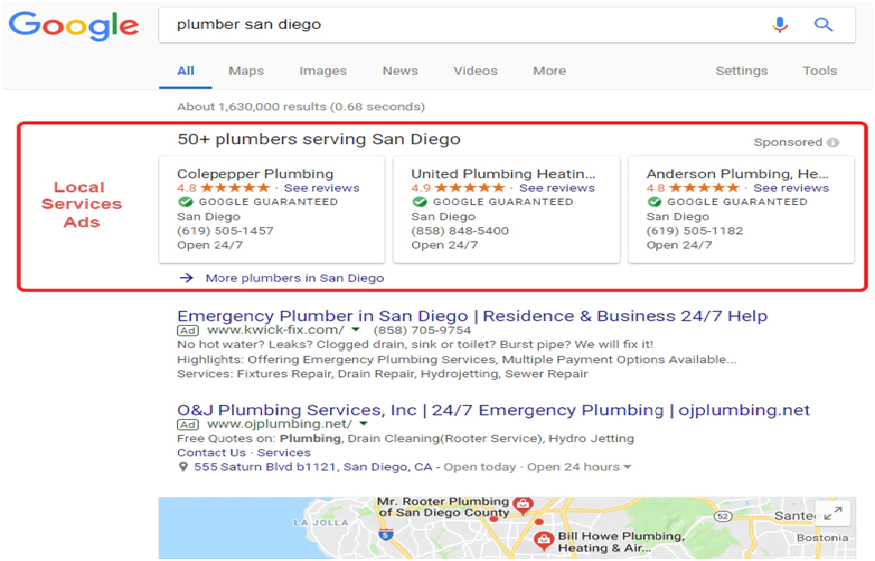### Descriptive Caption:

The image displays a Google search results page. At the top of the page, the Google logo is prominently featured, with each letter in the logo being colored distinctly: blue, red, yellow, blue, green, and red. Below the logo, there's a white search box situated against a gray background, which includes a blue microphone icon on the right and a blue magnifying glass icon to the left. The search query entered is "Plumber San Diego," typed in black text.

Below the search box, there is a horizontal menu with various tab options. The first tab, labeled "All," is highlighted in blue and underlined. The subsequent tabs, displayed in gray, are titled "Maps," "Images," "News," "Videos," "More," and "Settings & Tools."

Moving further down, the background changes to white, and there is a text line in gray stating "About 1,630,000 results (0.68 seconds)" indicating the number of search results and the time taken to generate them. This section is enclosed in a red rectangular border.

Within this bordered section, there is a red logo on the left. Below the logo, a black heading reads "50+ Plumber Service San Diego." The section showcases three outlined rectangles, each with information about a different plumbing service.

1. The first rectangle highlights "Cold Pepper Plumbing," with a rating of 4.8 stars and an option to "see reviews." It also has a "Google Guaranteed" badge.
2. The second rectangle features "United Plumbing," with a partial name display ("heap, ing..."), a rating of 4.9 stars, and an option to "see reviews."
3. The third rectangle mentions "Instant Plumbing" with a partial name display ("he..."), a rating of 4.8 stars, and an option to "see reviews."

Underneath these rectangles, there are two additional listings in a bluish color:
- The first one is "Emergency Plumber in San Diego," offering 24/7 help.
- The second one is "ONJ Plumbing Services, Inc.," also providing 24/7 emergency services, with a web address, "ojplumbing.net."